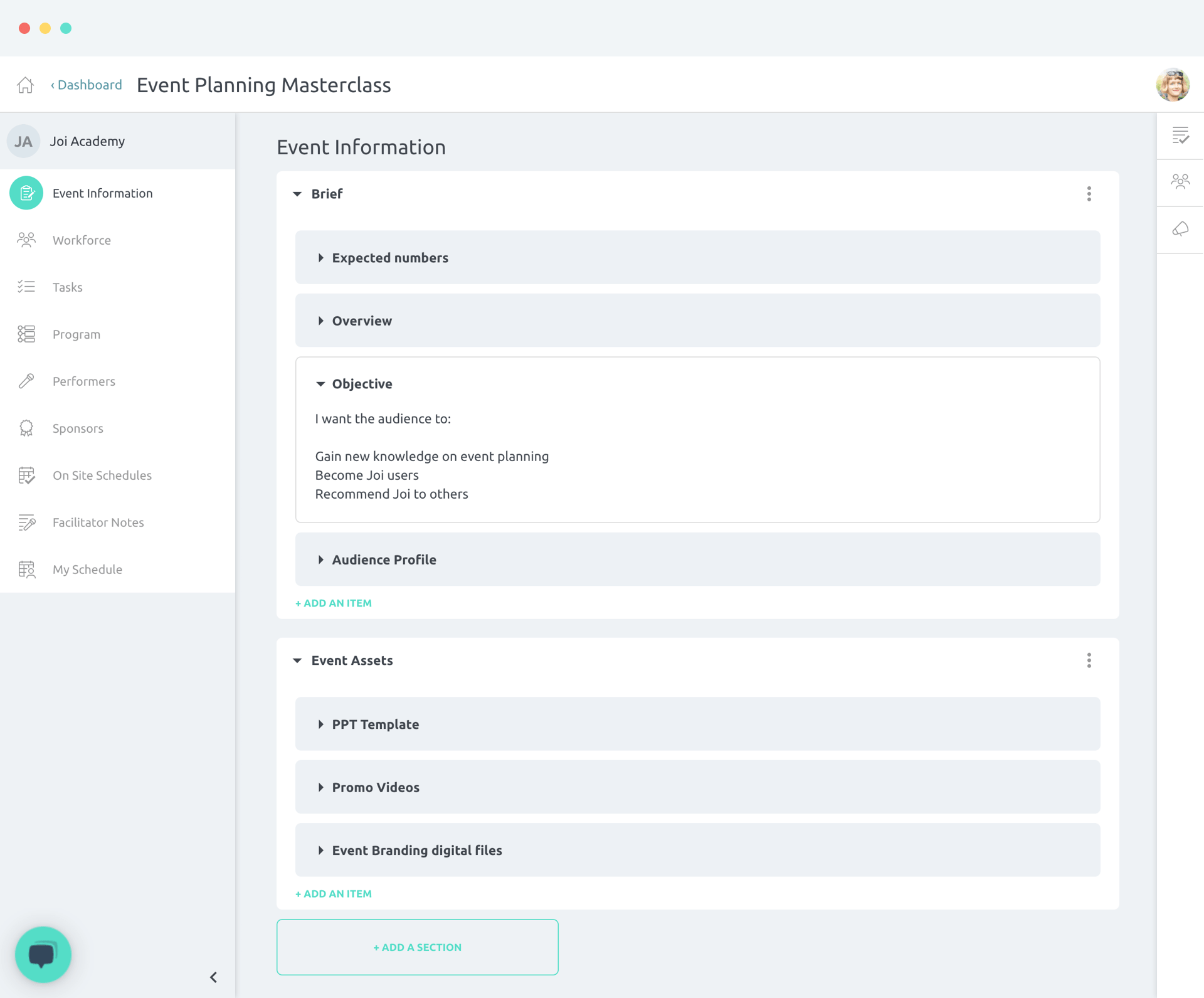This web page is designed for event planning and features a minimalist interface devoid of any images. At the top, there's a small icon resembling a home, which allows users to navigate back to the home screen. The page is titled "Event Planning Masterclass" prominently on the dashboard. 

On the left sidebar, under the label "JAJOL Academy," there is a vertical menu in black ink with several clickable options. The currently highlighted option is "Event Information," with additional menu items including Work in Force, Tasks, Program, Performers, Sponsors, Onsite Schedules, Facilitator Notes, and My Schedule.

To the right of the sidebar is a detailed view of the selected "Event Information" option. This section includes categories such as Brief, Expected Numbers, Overviews, and Objective—the latter being currently highlighted. The Objective section states the goal: "I want the audience to gain knowledge on event planning, become JOI users, and recommend JOI to others." 

Below the Objective, there are additional tabs that can be selected, namely Audience Profile and Event Assets. The Event Assets section lists items like PPT templates, promotional videos, and event branding digital files. Each item features a small triangle icon that can be clicked to reveal more information or options for adding items or selections.

Finally, located in the bottom left-hand corner of the screen, a small chat button is available for users who need additional assistance.